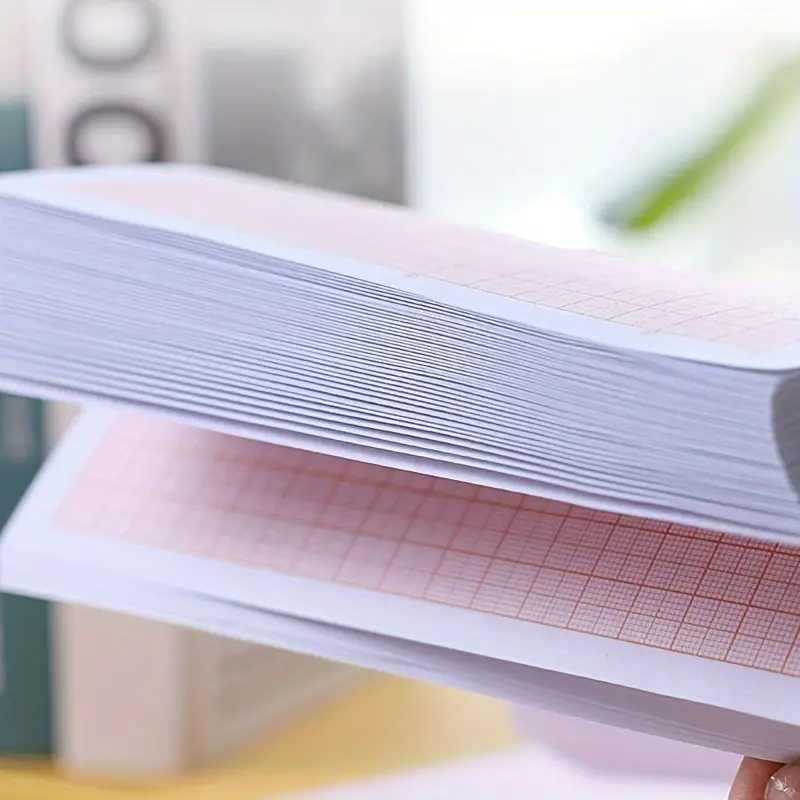The image features a detailed stack of graph paper, prominently displaying white pages with orange-red grid lines and a white border before the grids begin. The papers are divided into a thinner bottom stack and a thicker top stack, with a thumb and finger pulling down about ten sheets from the bottom right corner. This exposes the white edges and the grid lines beneath. The perspective is from the side, showing just a bit of the top of the stack. The background is notably blurry; however, a few elements can be discerned. On the left side, there's a book with a pink spine and a dark front cover, possibly black, displaying only the letter 'C' at the top. Additionally, there is a suggestion of a blue sky and a green plant coming down from the right corner, though these details are also out of focus. The overall setting hints at an indoor space, possibly a room in a house, but remains indistinct due to the blur.